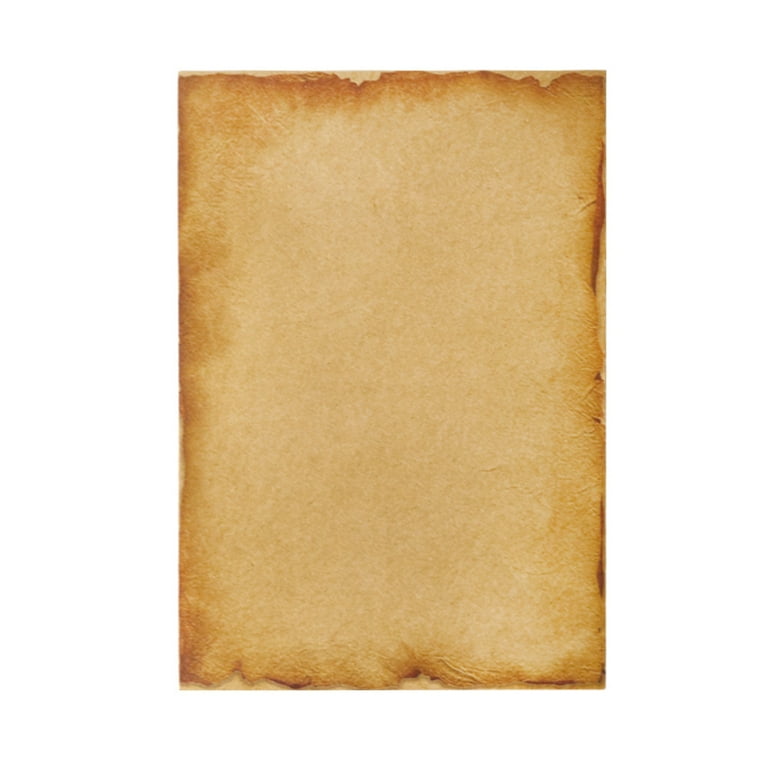This image features an aged, weathered piece of paper, exuding an aura of antiquity and historical significance. The paper, predominantly light brown in the center, transitions to a darker, almost charred appearance around its frayed and worn edges, suggesting prolonged exposure to the elements or perhaps a fire. The outer right edge is particularly affected, displaying a dense, dark brown hue that lightens gradually towards the middle. The bottom edge appears torn, with jagged, uneven segments and areas cast in shadow, enhancing the paper's distressed and mysterious character. The overall visual elements combine to tell a silent story of age, wear, and resilience.